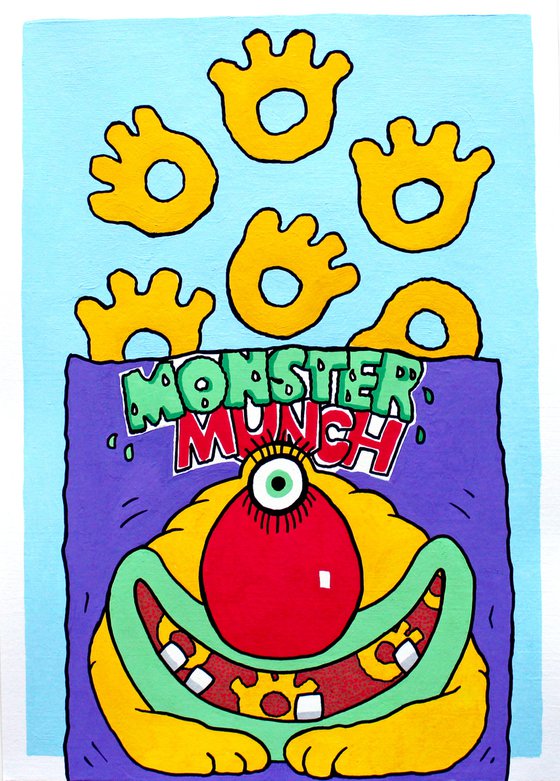The image is an illustrated artwork depicting a snack bag for a product called Monster Munch. The packaging is predominantly purple with the name "Monster Munch" prominently featured at the top, where "Monster" is written in green and "Munch" is in red with a thin white outline around the text. The background of the graphic is light blue, and all elements are outlined in black.

Central to the design is a whimsical, yellow monster. The monster has a single green eye with large eyelashes, a big red nose, and green lips forming a wide, crescent-shaped smile that seems to encompass most of its body. Inside its mouth, several yellow paw-shaped chips are depicted. The monster’s mouth, which is the size of its torso, also reveals four bottom teeth. The arms of the monster appear to be connected to its head.

Above the monster, chips that resemble animal paws - yellow with a circular base and four 'toes' at the top - are seen popping out of the bag. This character and the dynamic representation of the chips combine to create a playful and engaging snack package design.